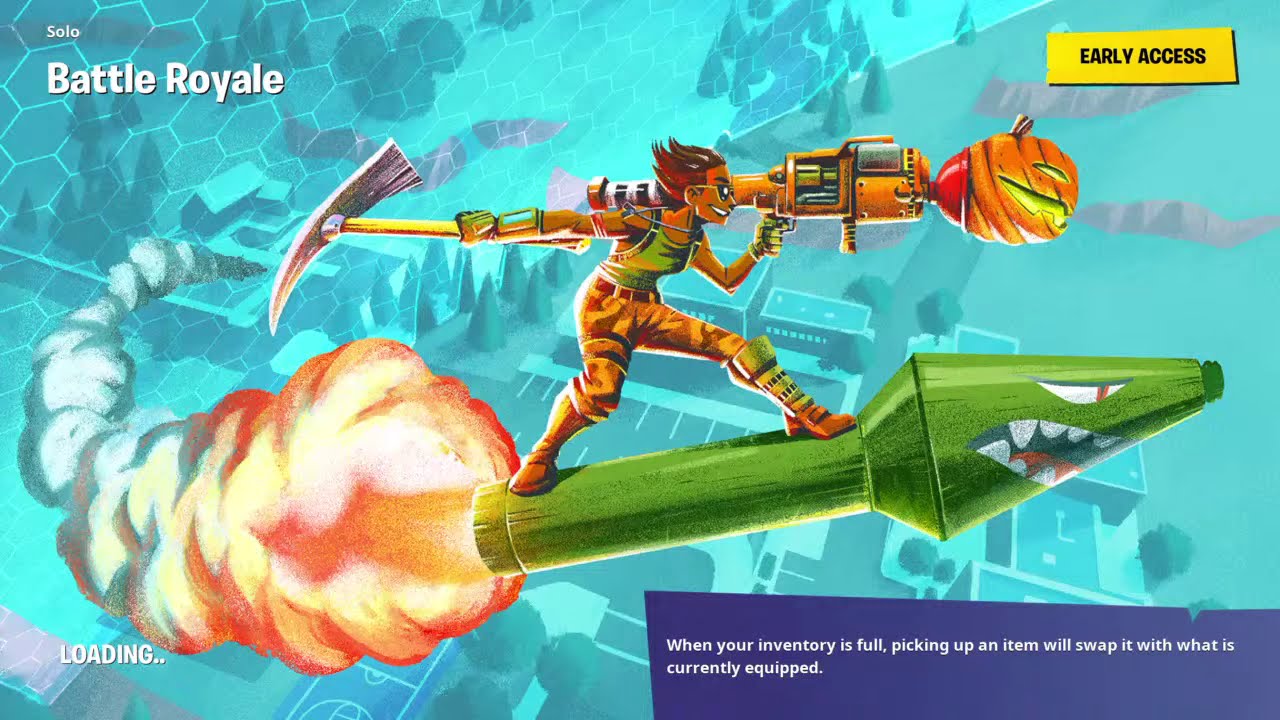This is an image from a video game featuring a woman dressed in a green tank top, brown and yellow camouflage pants, and boots, who is flying through the sky on a green rocket-like missile adorned with a cartoonish face, complete with white eyes and teeth. She is riding the rocket as if surfing, with a large gun resting on her left shoulder and a big chisel or pickaxe held behind her in her right hand. The rocket trails fire and smoke from its tail, with the smoke creating a visible path showing where it has come from. The background reveals an aerial view of a neighborhood with trees, buildings, and roadways. In the game's interface, "Battle Royale" is displayed in the upper left corner along with a honeycomb pattern, and "Early Access" is in the upper right corner. The lower left corner features the word "Loading," while the lower right corner contains the message, "When your inventory is full, picking up an item will swap it with what is currently equipped."